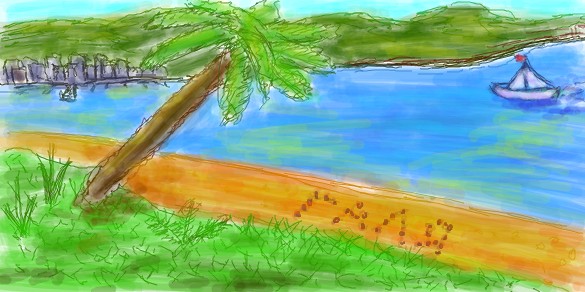This digital artwork, resembling a watercolor painting, features a serene island landscape. At the forefront, vibrant green grass seamlessly transitions into a sandy shoreline, which then meets the varying blue-green hues of the ocean. A prominent palm tree stands tall on the grassy area, its reflection hinting at the interplay of colors in the water below. Intriguingly, an arrangement of rocks spells out an indistinct message in the sand, possibly reading "R-A-A-R." A small white sailboat with a distinct red flag is seen calmly anchored in the azure waters. In the distance, lush green mountains rise, completing this tranquil, nature-rich scene dominated by verdant tones.